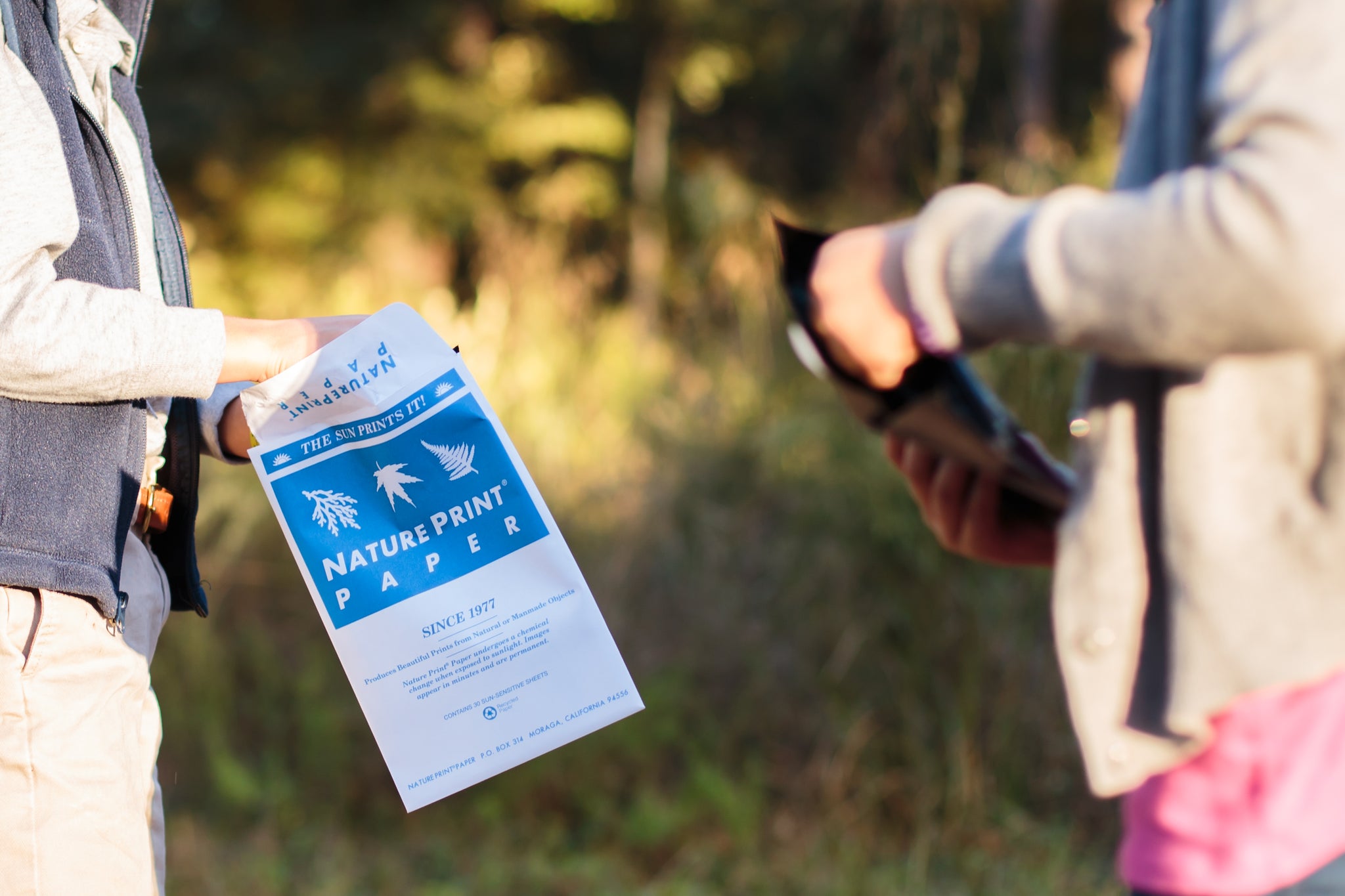The photograph, taken outdoors during the daytime, is rectangular in shape, approximately five inches wide and four inches high. It features two people standing amidst a blurry backdrop of green grass and foliage. The man on the left is visible from mid-thigh to collarbone, dressed in light brown pants and a matching long-sleeve shirt, over which he wears a gray fleece vest. His hands, bent at the elbows, are obscured by a rectangular white bag that he holds, prominently displaying a blue square with white print that reads, "Nature Print Paper since 1977," adorned with images of leaves. To the right, a slightly shorter individual, visible from the mid-thigh to shoulder, wears a long-sleeve light brown jacket over what appears to be a pink shirt. This person's arms are also bent at the elbows, facing the man on the left, and seem to be holding another similar bag, although it is shadowed and blurred, making the details less distinguishable. The background of trees and brush is also blurry, indicating that the focus is primarily on the two individuals and the objects they are holding.